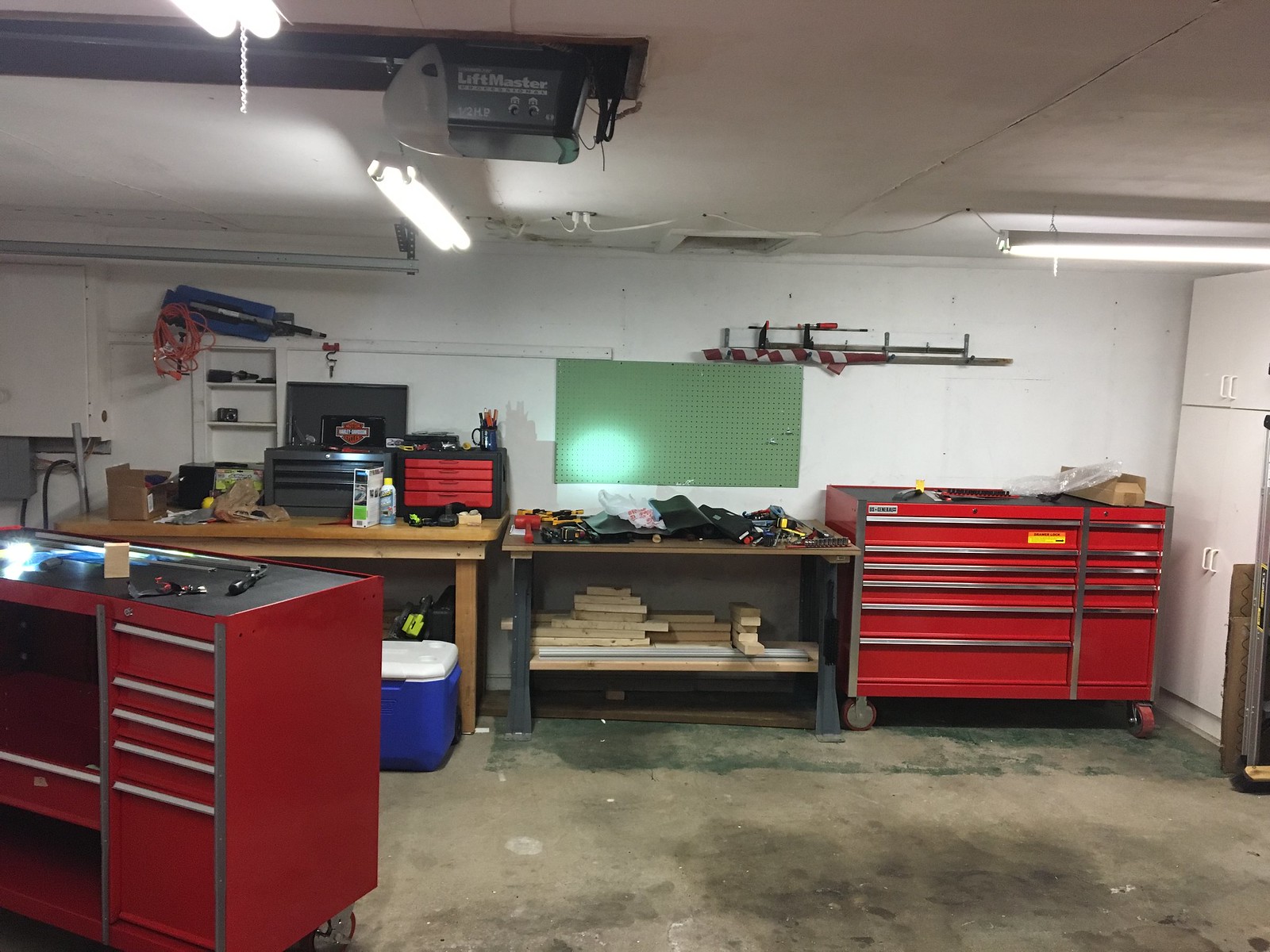This image captures the interior of a garage or wood shop, featuring a gray cement floor with various black stains. Prominently, there are two bright red storage containers with silver detailing on their drawers; one positioned in the left-hand corner and the other against the right side of the garage. The red storage containers are likely tool chests, with one even sitting on a cart. 

A white cabinet with corresponding white handles stands next to the right-hand tool chest. In the center of the space, multiple workbenches are cluttered with tool bags, piles of wood, and other planning materials. A brown wooden table holds containers with small red and black drawers, likely for organizing smaller items or tools. 

Along the wall, a rolled-up American flag is visible, though not fully displayed. Above one workbench, there is a green pegboard, notably devoid of any hanging tools. The ceiling features hanging fluorescent lights and the tracks for the garage door, with a projector mounted near the top. A partially obscured white and blue cooler is tucked near one of the red tool chests, adding to the functional yet cluttered environment.